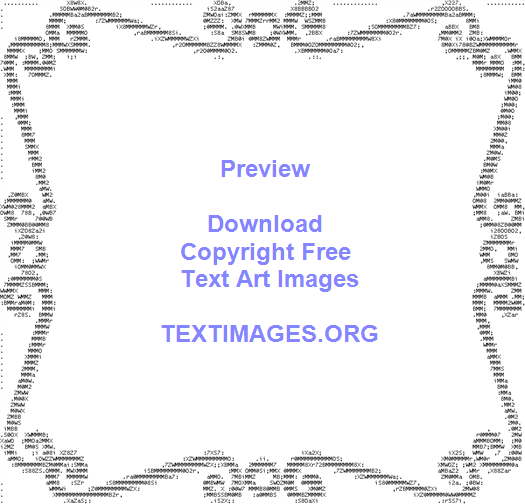The image features a white background with an intricate, classical frame made up of interwoven black text characters, numbers, and letters, giving it a nostalgic, scroll-like appearance. The text within the frame is displayed in light purple and is arranged in three lines: "PREVIEW" at the top, "Download Copyright-Free Text Art Images" in the middle, and "TextImages.org" at the bottom, all in uppercase letters. This intricate design combines the aesthetic of vintage labels with modern digital elements, suggesting an advertisement for a website offering free downloadable text art images.